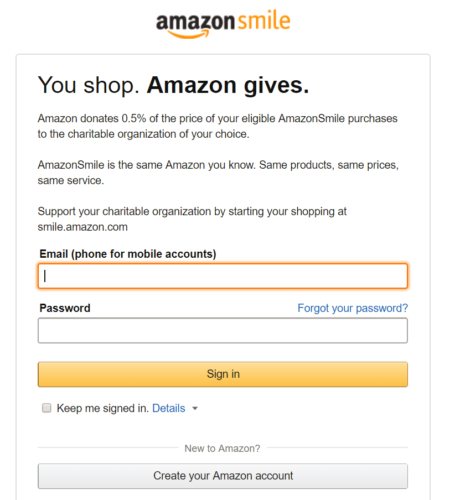The image is a screenshot of a portion of the Amazon Smile website. At the top, the logo reads "AmazonSmile," followed by the tagline: "You shop. Amazon gives." The text continues to explain that Amazon donates 0.5% of the price of eligible purchases to a charitable organization of the user's choice. This donation program is part of Amazon's service and maintains the same products, prices, and customer service as the main website. The message encourages users to support their favored charitable organizations by shopping through smile.amazon.com. Below this explanatory text, the image features a typical login section. The first text box is labeled "Email" (with "phone for mobile accounts" noted in parentheses), and the second text box below it is labeled "Password."